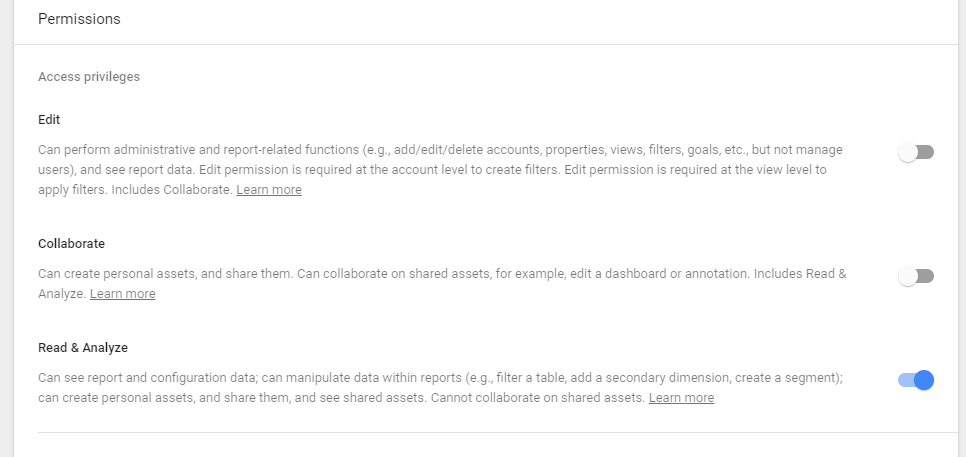In the screenshot provided, we see a user interface clearly designed for setting up and managing the functionalities of a website. The interface is structured to control various permissions and access levels. At the top-left corner, the word "Permissions" is prominently displayed, indicating the section's purpose.

Below "Permissions," there is a faint horizontal line serving as a separator. The section is further divided into three distinct categories, each with a toggle switch to the right that allows the user to activate or deactivate the corresponding permissions.

1. **Edit**:
   - **Description**: This category highlights the user's ability to perform a range of administrative and report-related functions. Specifically, users can add, edit, and delete accounts, manage priorities, views, filters, and goals, among other tasks.

2. **Collaborate**:
   - **Description**: Users granted this permission can create personal assets and share them. They can also collaborate on assets that are shared with them.

3. **Read and Analyze**:
   - **Description**: This category outlines the user's access to viewing and analyzing data. This is the only permission currently enabled, indicated by the blue toggle switch to its right.

Each permission category is distinctly marked with bold lettering to emphasize its significance, making it easier for users to navigate and understand the functionalities they are managing.